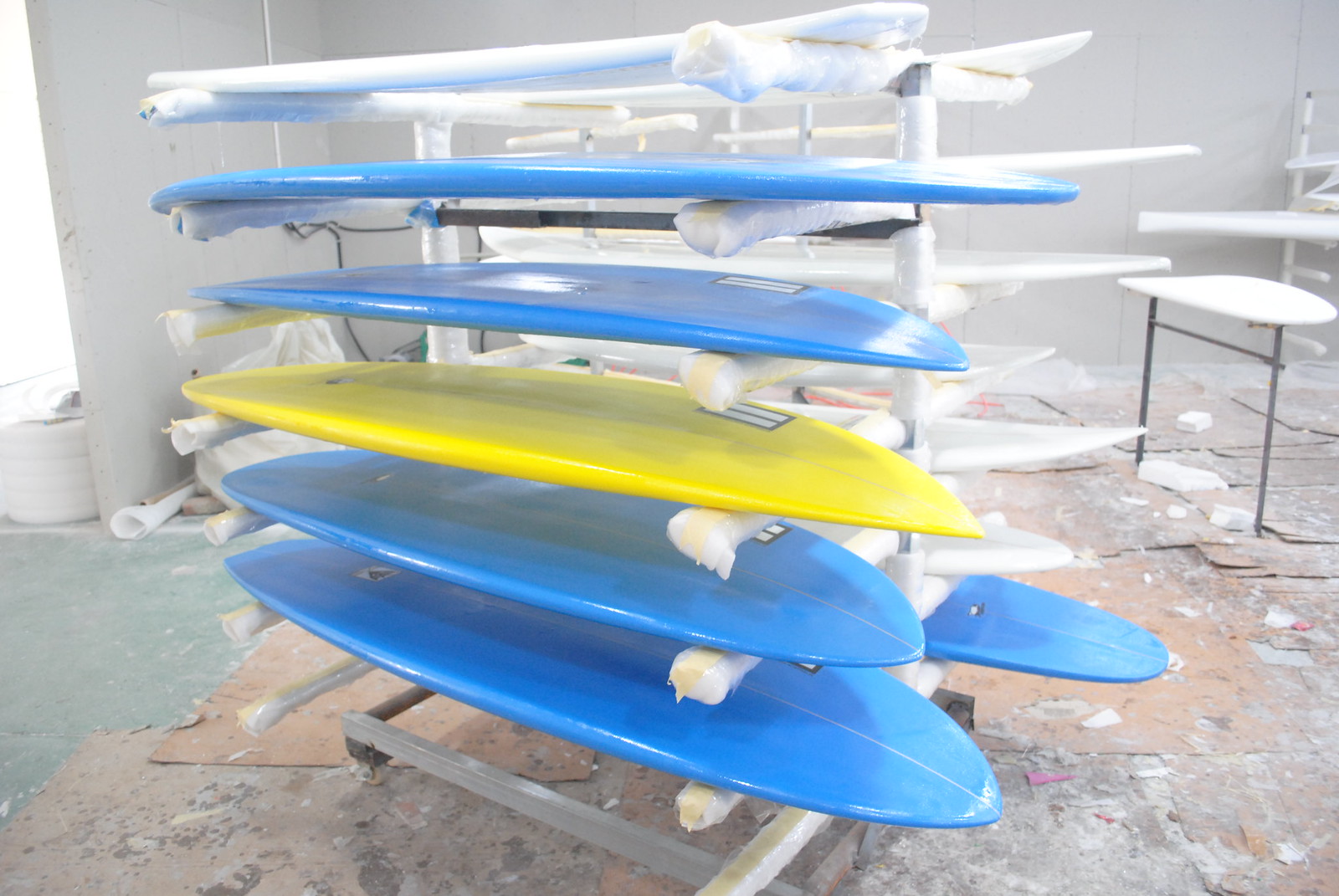The image depicts around thirteen to fourteen freshly painted surfboards organized on white padded racks. The surfboards feature various colors: three are a rich royal blue, one stands out with a pointy yellow tip, and the remaining are all white. The surfboard holder appears to be a rolling cart with arms extending for placing the boards on both sides. This setup is situated in what looks like a warehouse, characterized by a grayish wall in the background and a notably decrepit floor. The floor is cluttered with paint splotches and strewn with brown sheets of cardboard, adding to the general messiness of the area. There is also a small white table to the side, likely used for surfboard work. The overall environment appears run-down, with a concrete floor that looks shattered and unsafe for walking barefoot. In the back right-hand corner, another stack of boards can be partially seen, adding to the disarray of the space.